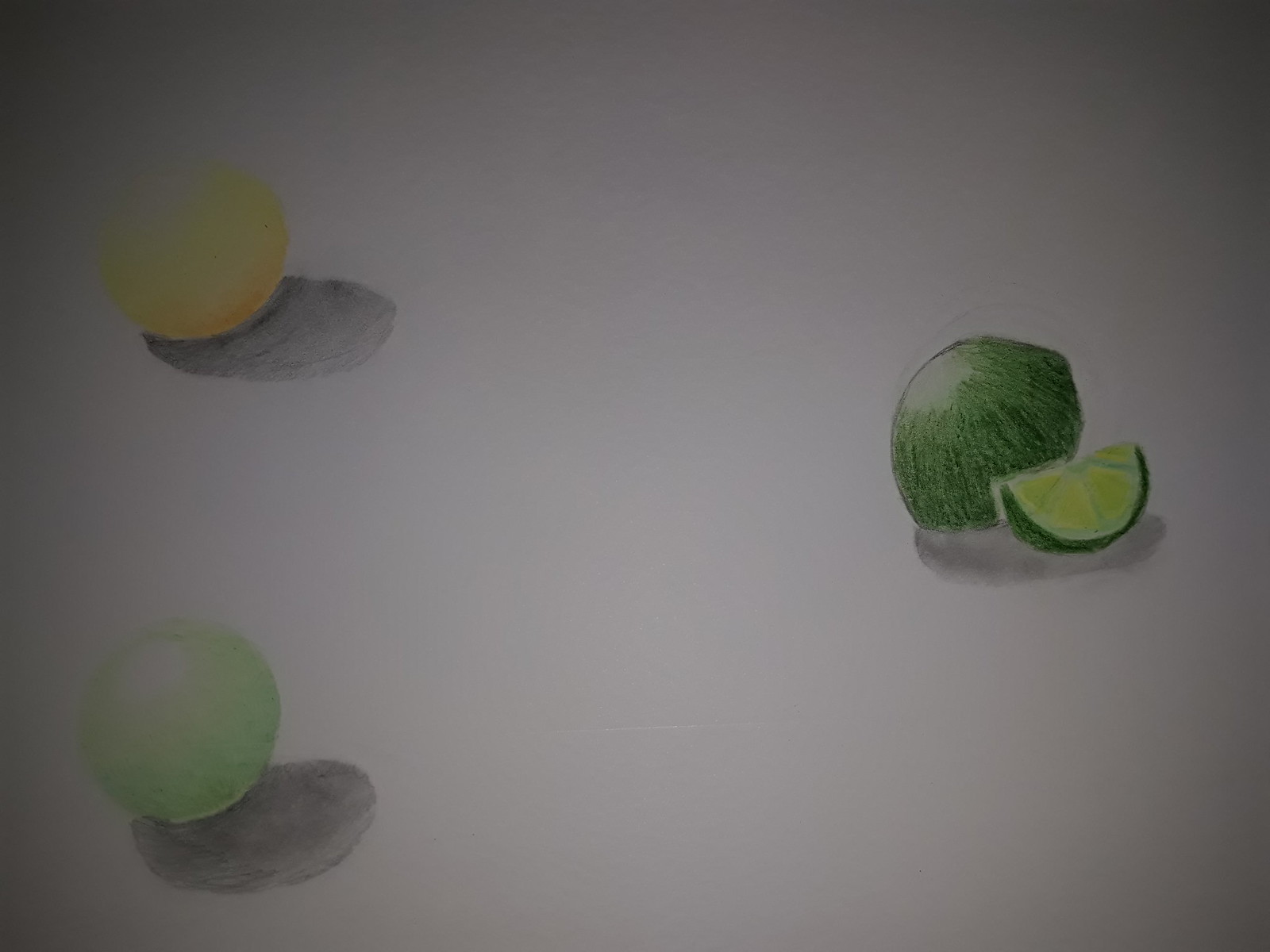This hand-drawn image, rendered with colored pencils, showcases three distinct fruits meticulously arranged against a light grey background, reminiscent of snooker balls spaced apart on a table. On the left, there's a whole green lime, accompanied by a sectioned wedge, revealing its yellow-tinged interior and a white splotch in the middle. The lime casts a gradient shadow starting from dark grey under the fruit, gradually lightening outward. On the right side of the paper, a vibrant lemon, transitioning from a light yellow at the top to a deeper hue at the bottom, similarly leaves a distinct dark to light grey shadow beneath. In the bottom left corner, a Granny Smith apple is drawn with a striking gradient – predominantly green at the bottom morphing to a yellowish tint at the top, also casting a dark shadow. The interplay of colors and shadows gives the drawing depth and realism, capturing the essence of each fruit against the subtly grey-toned background.